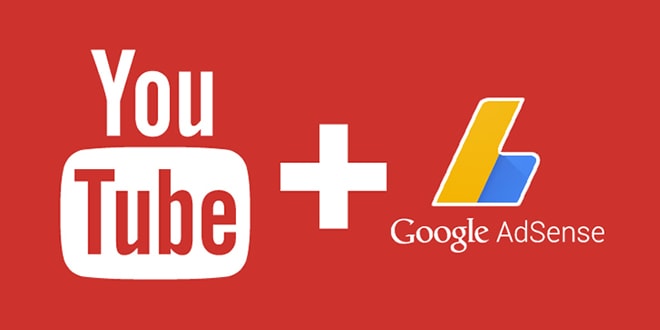The image features a red sign prominently displaying the YouTube and Google AdSense logos. The YouTube logo is composed of the word "You" in white letters, while "Tube" appears in red letters set against a white background. Beside it, there is a white "+" sign, indicating a collaborative relationship. Adjacent to the plus sign, the Google logo is presented in its iconic multi-colored lettering, followed by the words "Google AdSense" in a straightforward black font. This sign likely symbolizes the integration of Google AdSense with YouTube, suggesting a partnership where Google provides advertising solutions for the video platform.